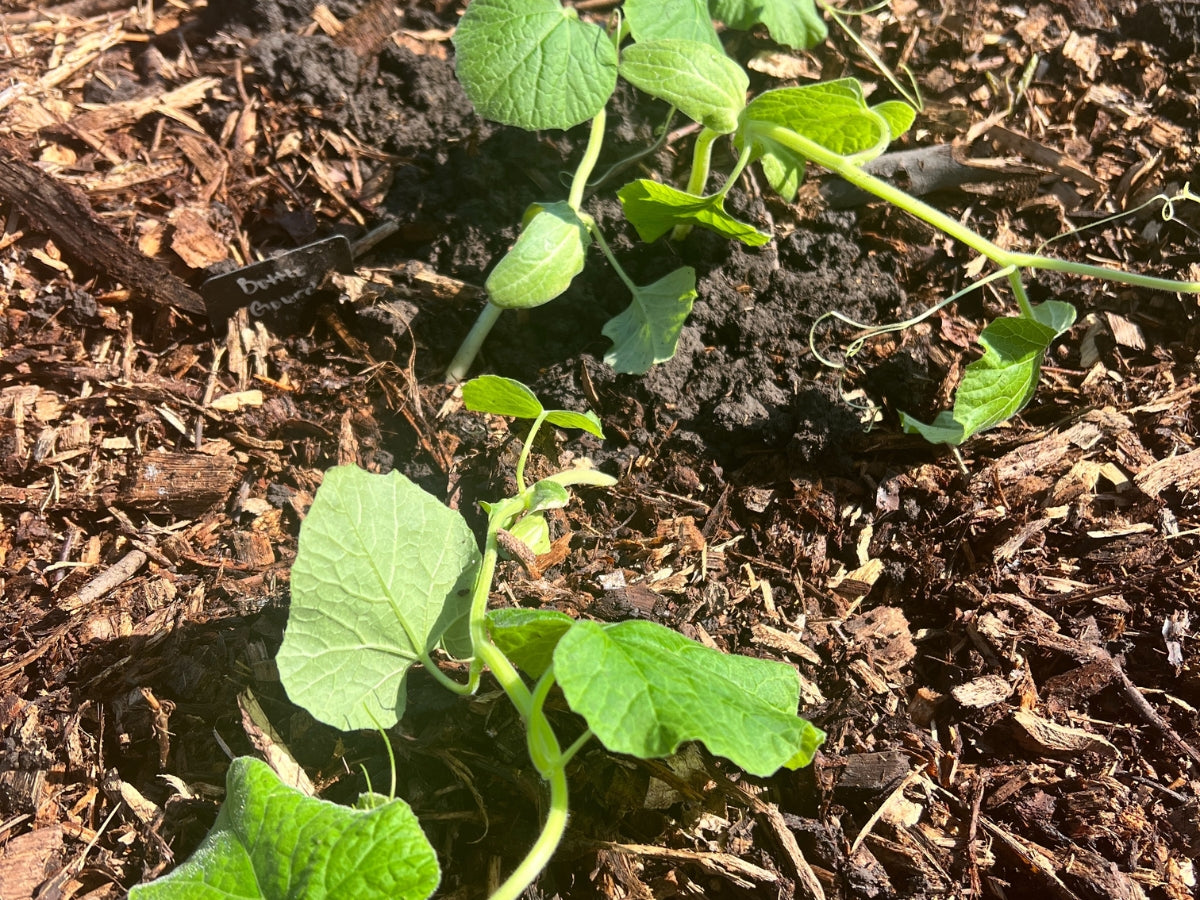This close-up, rectangular photograph captures vibrant green bottle gourd sprouts emerging from a small soil pocket surrounded by light brown wood mulch. The image, illuminated by natural sunlight, details the fresh, spring-green heart-shaped leaves of the sprouts, with their veins prominently visible from this proximity. In the background, dirt is interspersed with chunks of mulch. A small metal label, placed near the plants, clearly reads "bottle gourd," indicating the type of plant. The young bottle gourd leaves resemble those of a pumpkin, and some tendrils are just starting to spread from the plants, which are in their early stages of growth.